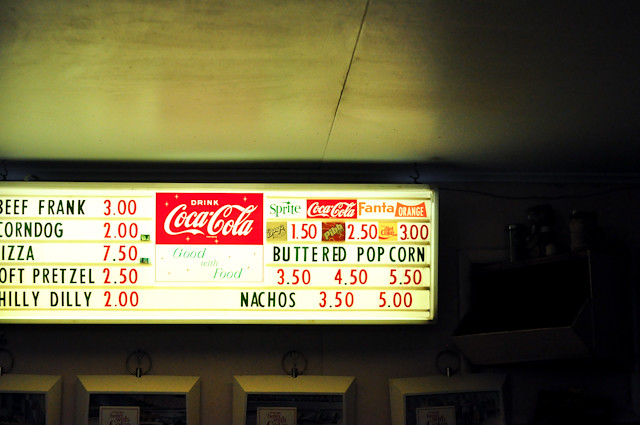The image depicts a brightly lit menu sign at a concession stand, likely situated in a movie theater. Below this illuminated menu are four sleek, silver display cases with ring-like handles on top and glass fronts, hinting at contents stored within. The menu sign is the focal point, featuring a series of food items listed in black uppercase text, while the prices are highlighted in red. 

The offerings include:
- Beef Frank: $3
- Corndog: $2
- Pizza: $7.50
- Soft Pretzel: $2.50
- Philly Dilly: $2
- Buttered Popcorn: $3.50, $4.50, $5.50
- Nachos: $3.50, $5

The sign also prominently displays the Coca-Cola logo accompanied by the slogan "Drink Coca-Cola" and another phrase "Good with Food" in green writing. Beverage options are illustrated with their respective logos and prices, including:
- Sprite
- Coca-Cola
- Fanta Orange
- Mr. Pibb: $2.50
- Diet Coke: $3
- Barq's: $1.50

The image is horizontally oriented, providing a view of the white ceiling above the menu. The concession stand itself is less visible due to the intensity of the sign's light, which dominates the scene, leaving much of the area below the menu in shadow except for the glint of the silver cases.